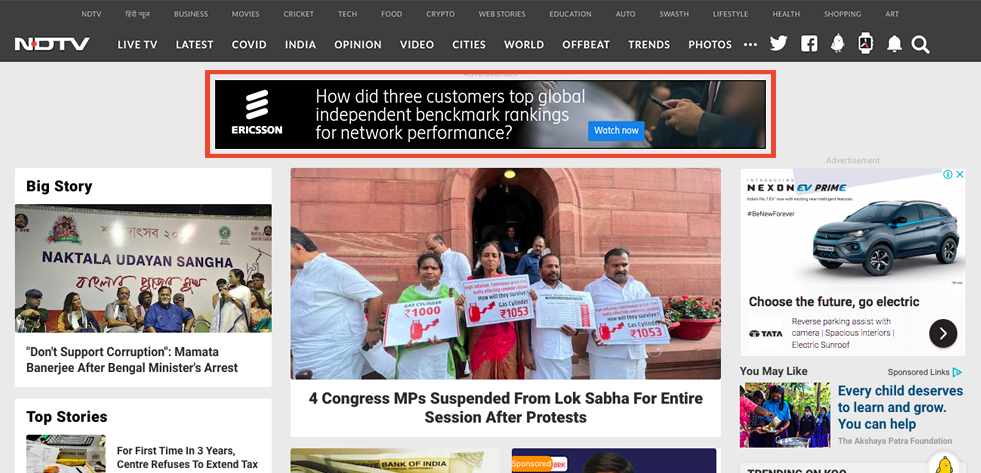Here's a thoroughly detailed and cleaned-up caption for the described image:

"This vibrant collage encapsulates multiple facets of modern life and media, highlighting an array of categories including Business, Movies, Cricket, Tech, Food, Crypto, Webstores, Education, Auto, Lifestyle, Health, and Shopping, all represented under the NDTV banner. Prominent icons for live streaming, latest news updates, Covid information, and regional sections like India, Cities, and World are prominently featured. Social media icons for Twitter and Facebook, along with symbols for notifications and search, are also visible.

Incorporated in the design is a key update: three customers achieved top positions in a global independent benchmark ranking, marked by the numeric 4 and a question mark, with Ericsson being prominently mentioned. The layout features a blue border in the bottom right cautioning users to avoid interference with smartphone navigation. Surrounding elements include a thin white border, followed by a thicker red border.

Additional headlines capture immediate attention, such as 'Big Story' and 'Naktala Udayan Singhao'. A firm stance against corruption is urged following a Bengal minister's arrest. The 'Top Stories' section is followed by 'Next Song Evie Prime', promoting electric vehicles with highlights on futuristic design, spacious interiors, parking assistance with cameras, and electric sunroofs. A prominent call-to-action stresses, 'Every child deserves to learn', hinting at an educational initiative or campaign."

This caption provides a thorough and clear description of the image, incorporating all visual and textual elements mentioned.